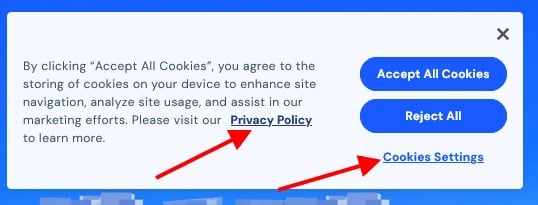The image depicts a pop-up box commonly seen on websites, prompting users to manage their cookie preferences. The background is a gradient of blue, providing a calm and professional context. At the center of the image, there is a clean, rectangular white box containing several actionable elements. 

At the top of the box, there is a headline that says "Privacy Policy," inviting users to click on a link to read the website’s detailed policy on cookies. Below the headline, there are three primary options for the user:

1. A blue button labeled "Accept All Cookies" located centrally towards the right.
2. Directly beneath it, another blue button labeled "Reject All Cookies."
3. An underlined blue text link labeled "Cookie Settings," positioned below the aforementioned buttons, offering users a chance to customize their cookie preferences.

There is a small space separating these options for clarity and visual hierarchy. Additionally, on the left-center, a descriptive text explains, "By clicking 'Accept All Cookies,' you agree to the storing of cookies on your device," ensuring that users understand the implications of their choices. The overall layout is user-friendly, guiding the user through their privacy options effectively.